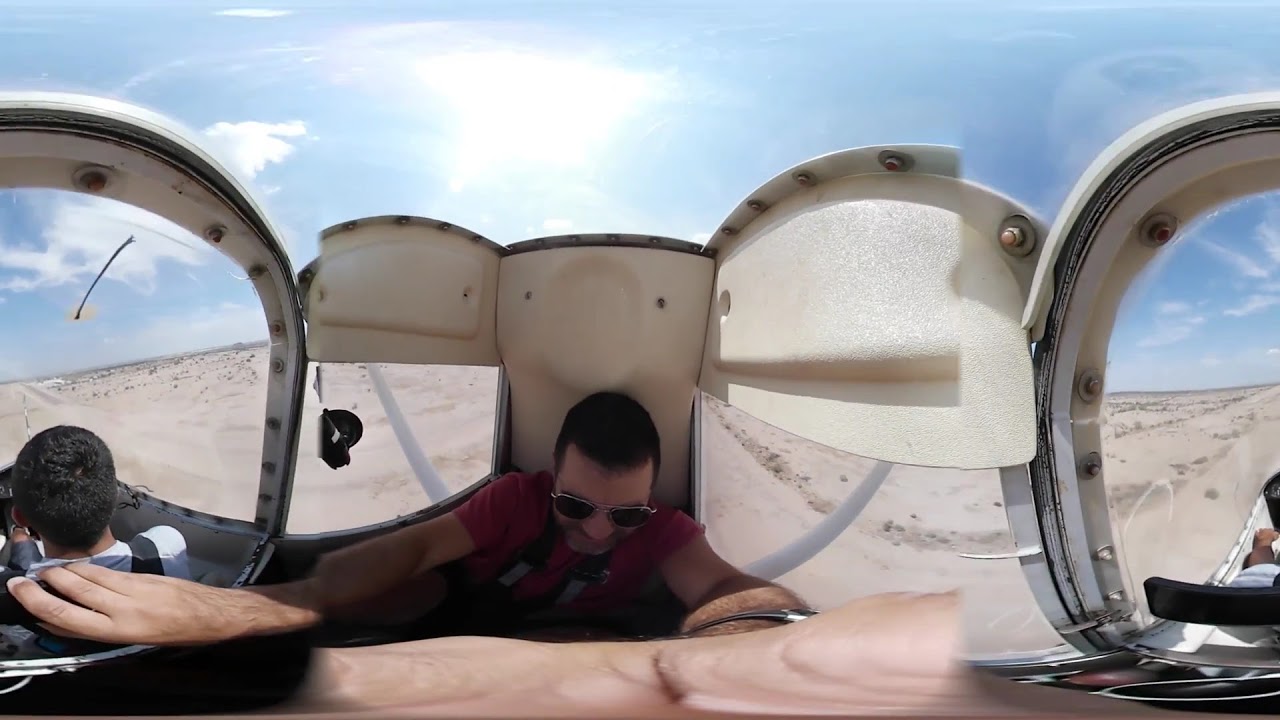An outdoor color photograph captures a man sitting in the cockpit of an open-air, likely light aircraft or vehicle parked in a sandy, possibly desert location under a bright, blue sky adorned with puffy white clouds. The man, who appears to be Caucasian with dark brown hair, is wearing dark aviator sunglasses and a red t-shirt. He is looking down at an instrument panel, with his right arm more prominently extended than his left, suggesting interaction with the cockpit controls. To the left, part of another person is visible, a young individual with dark hair wearing a white t-shirt and a safety strap, indicating they are securely seated. The curvature of the vehicle’s fiberglass or plastic windows is evident, framing the view of a flat horizon line with a paved road or runway extending into the distance. A glimpse of another potential passenger is visible on the far right, obscured by the crop of the photograph. The setting sun casts a bright patch of light across the scene, enveloping the activity in a sunny, open, and somewhat arid environment.